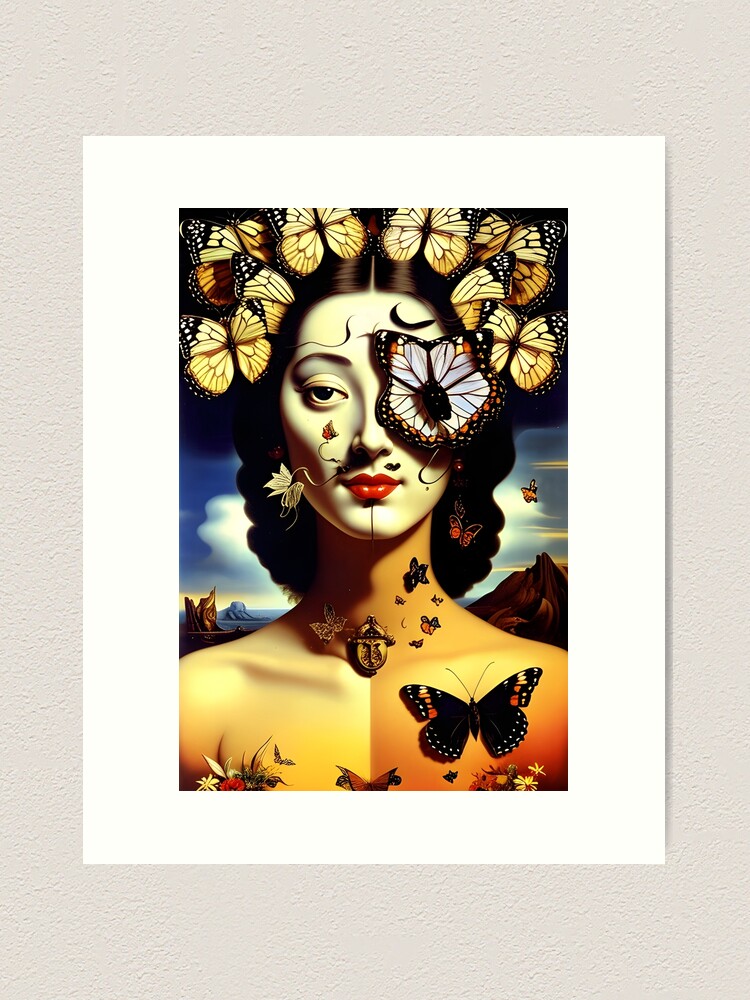This detailed digital illustration showcases a central figure of a woman from just below the neck up, with contrasting skin tones on either side of her body. Her untanned, lighter side contrasts with the darker, tanned side, emphasizing an artistic expression of duality. The woman's face is adorned with intricate makeup, and her head is surrounded by a swarm of vibrant butterflies, with one butterfly covering her eyebrow and eye on one side. Above her head, approximately eight to ten butterflies obscure much of her hair, while around six butterflies are scattered near her shoulder and chest. The background hints at a surreal landscape featuring mountains, a river or lake, a streaked sky, and clouds. This striking image, rendered in pen and ink with vivid colors and fine detailing, appears to be a digital replication of a poster, with a white border and a light gray background. No watermarks or signatures are present, enhancing the focus on the fantastical elements surrounding the woman.